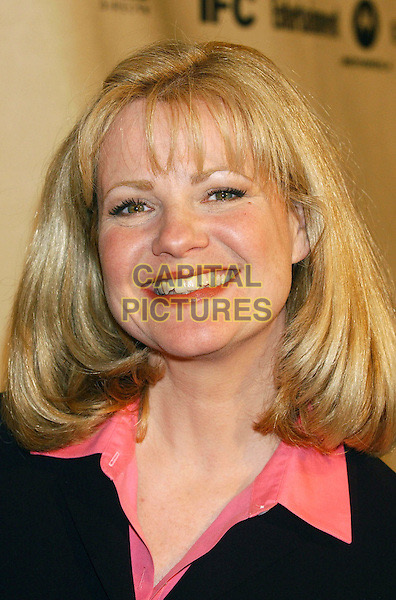This photograph captures a smiling blonde woman with shoulder-length hair and bangs, giving off a friendly and warm-hearted vibe. Her complexion is rosy, and she wears red lipstick and possibly mascara, highlighting her greenish-brown eyes. The woman is dressed in a bubblegum pink collared button-up shirt, which is open at the top, under a black sweater or blazer. The image features a visible watermark in light gray with a yellow border that reads "CAPITAL PICTURES" in all capital letters. In the background, there is a wall with some printed text, including the word "IFC," suggesting the setting might be related to the television channel. Her head is slightly tilted to the left, adding a touch of charm to her open and inviting facial expression.